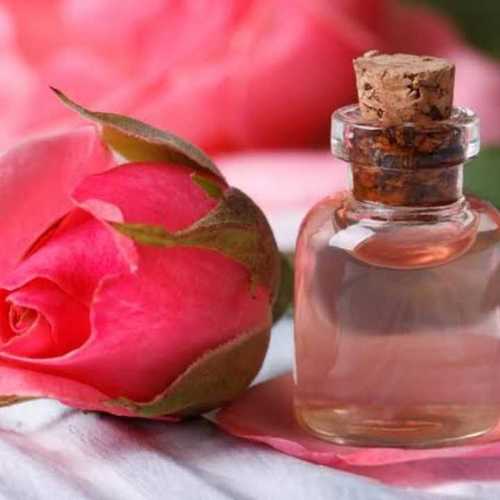This is a detailed close-up photograph featuring a delicate composition of a small glass bottle and a rose. The small bottle, positioned on the right, is crafted entirely from clear glass and is sealed with a cork stopper. It contains a clear liquid that appears to be water but could be another substance like alcohol. The bottle is diminutive, with an elegant, curving shape that converges at the neck before flaring slightly at the mouth, held closed by the cork.

To the left, partially lying across a slightly wrinkled, white fabric surface—possibly cloth or paper—is a reddish-pink rosebud. The rosebud's green leaves are visible on the outside, adding a fresh contrast to the scene. The rose is oriented at a gentle angle, with the bud closer to the left side of the frame and the stem stretching toward the right. Beneath the bottle, there is a pink object that appears to be a rose petal, enhancing the delicate nature of the arrangement.

The background of the photograph is soft and out of focus, subtly hinting at additional pink elements—likely more flowers—that add a dreamy and cohesive atmosphere to the composition. This careful interplay of elements and textures creates a harmonious and aesthetically pleasing image.